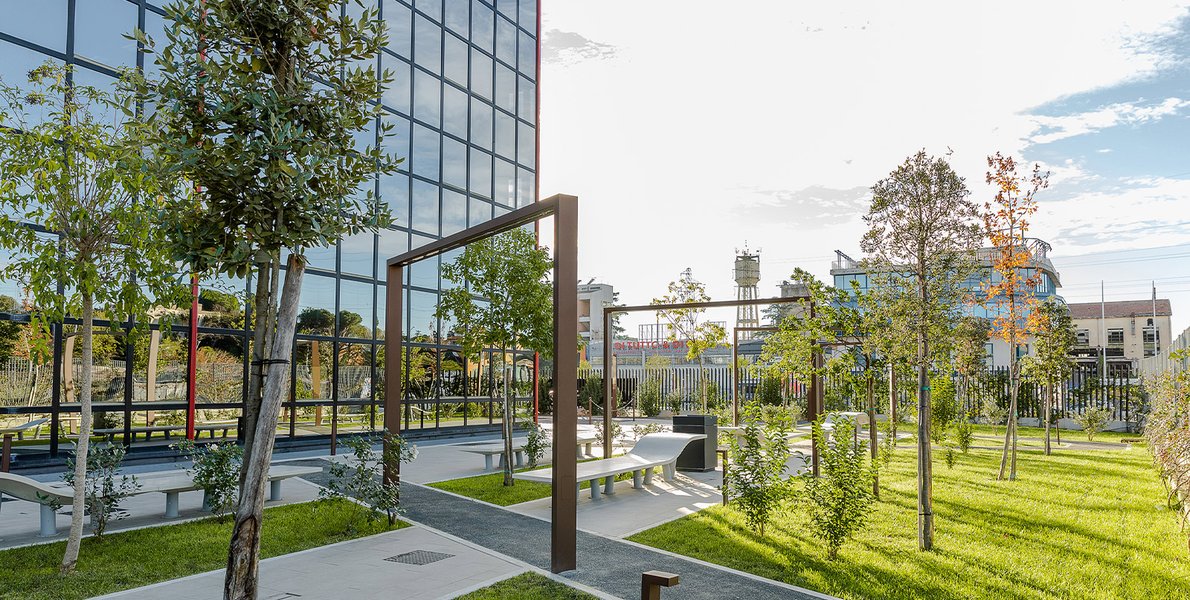This color photograph captures a modern urban scene dominated by a tall, mirrored building on the left side, whose reflective surface beautifully mirrors the surrounding trees and overcast sky. In front of this building, a row of lush green trees adds a touch of nature to the sleek, architectural setting. Centrally positioned in the image are two tall brown metal archways, which frame a long, white bench, inviting passersby to sit and relax. A dark gray pathway cuts diagonally across the scene, guiding the viewer's eye through the composition. To the right, a green grassy area with additional trees provides a soothing contrast to the built environment. In the background, glimpses of other buildings and a prominent tall water tower are visible. Overall, the image presents a harmonious blend of urban design and natural elements under an overcast sky, with no legible writing to distract from the visual narrative.